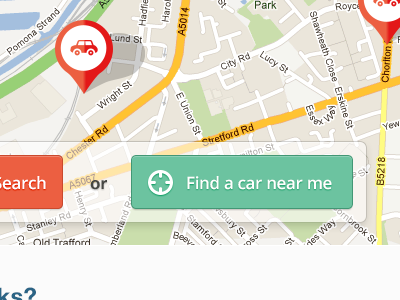The image appears to be a screenshot from a mapping application or website, featuring a highly detailed, zoomed-in view of a specific area. The map itself has a gray base color, with white streets and roads, while certain roads marked with yellow likely indicate larger roads or highways. Street names visible include "City Road," "Lucy Street," and "East Union Street."

Overlaying the map is a translucent rectangular box housing two interactive buttons—one red and partially visible with the text "E-A-R-C-H," likely indicating a "Search" function, and a green button labeled "Find a Car Near Me." There are also two red and white location markers with car icons, suggesting designated car locations or points of interest related to car services. The detailed nature of the map indicates close proximity to these locations, making it clear and easy to identify specific streets and their connectivity.